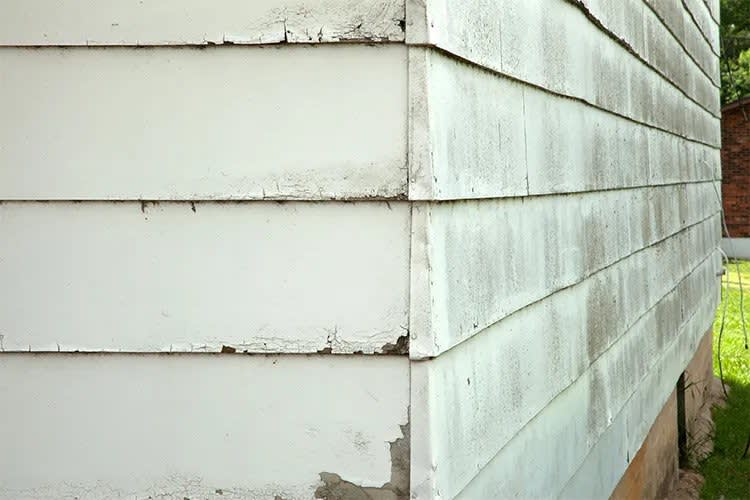The image captures the weathered corner of a wooden house, emphasizing the deteriorated state of its white paint. The flaking paint reveals grey wood underneath, especially pronounced at the bottom, highlighting the need for a fresh coat. The house siding comprises ten rows of horizontal boards on the right and four on the left. The right side of the house appears notably dirtier, with visible brownish-grey stains and white cords emerging from the wall, suggesting possible electrical or cable lines. Below the siding, the foundation, possibly made of brown stone or wood, hints at structural sturdiness despite the visible wear and tear. A patch of sunlit, bright green grass encroaches on the lower right corner, contrasting with the aged facade. In the background, a red brick wall and green trees partially visible above add color and depth to the scene, further highlighting the house’s rustic charm amidst its need for maintenance.